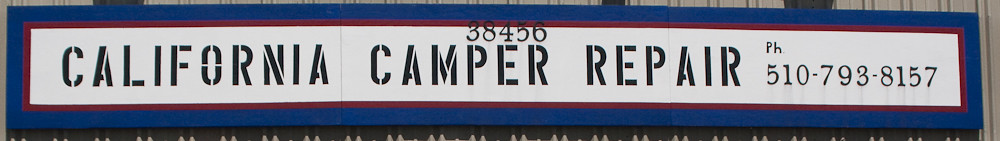The tightly cropped horizontal strip color photograph depicts a large sign prominently displayed atop a metal corrugated building or shed. The sign features a white background at its center, encased first by a thin red border and then a thicker blue border. Boldly spanning the center of the sign is stencil-style capital letter text spelling out "California Camper Repair." To the right of the main text, "PH" is printed, followed by a phone number below it, "510-793-8157." Additionally, at the center of the sign, overlapping the red and blue borders above the letters "PER" in "Camper," is a smaller, black text that reads "38456." This detail adds an extra layer of specificity to the otherwise straightforward advertisement for the camper repair service.